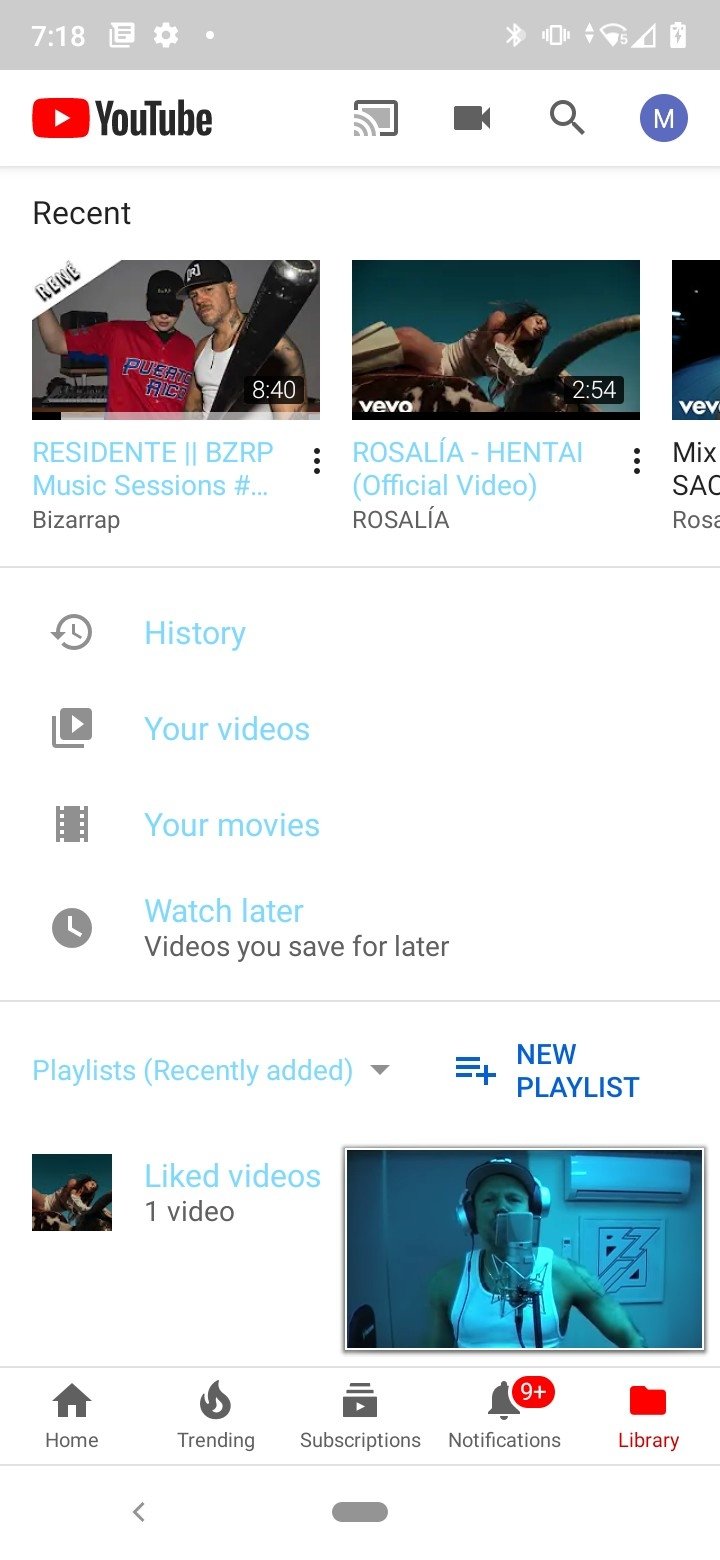In this image, we observe a screenshot. The upper left corner, set against a gray header, displays the time "7:18" in white text. Adjacent to this is the icon for settings. The upper right corner features white icons indicating Bluetooth, Wi-Fi, reception strength, and battery status. 

Below, on a white background, the upper left corner reads "YouTube" in black text, accompanied by the YouTube icon—a red rectangle with a white play button in the center. To the right of this, there is a blue circle containing the letter "M," representing the user's ID.

Further down, in gray text on the left side, appears the word "Recent". Two video thumbnails are displayed below this heading. The first thumbnail reads "Resident Music Sessions" in blue text. To its right, the second thumbnail reads "ROSALÍA - HENTAI (Official Video)".

Additionally, in the left margin, blue text reads vertically, listing options as follows: "History," "Your videos," "Your movies," and "Watch later."